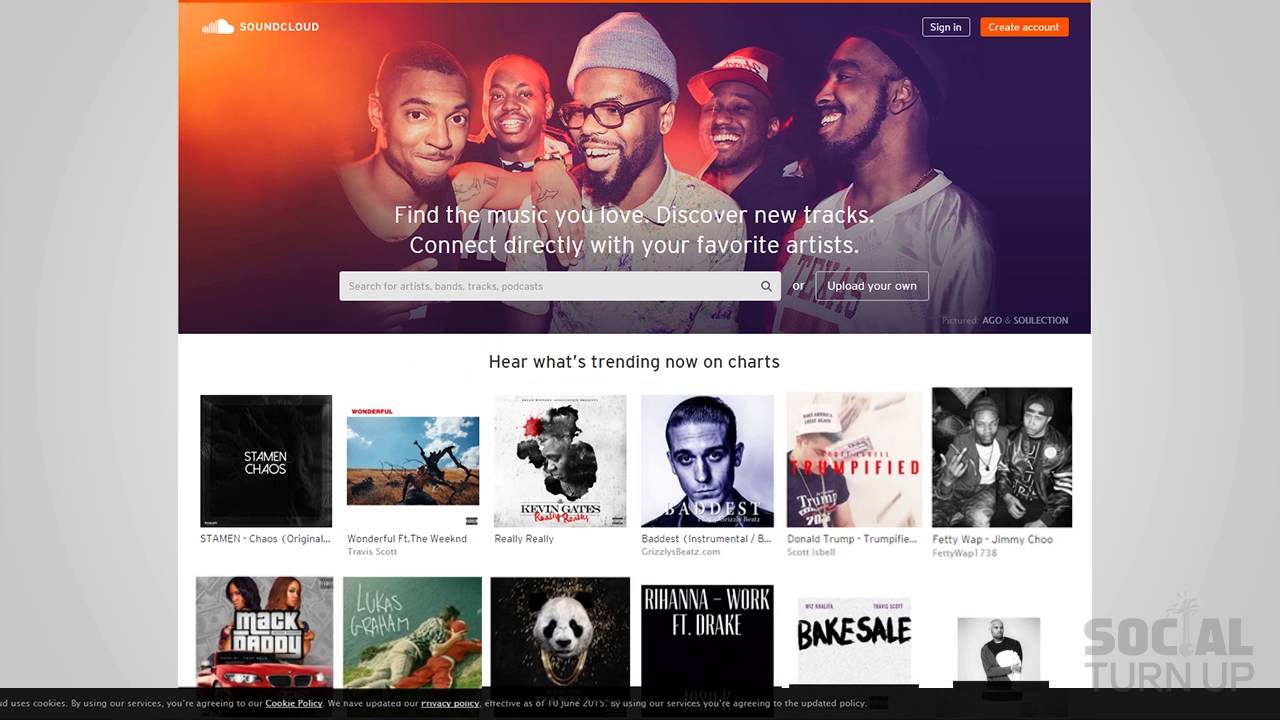The image consists of a large gray rectangle, inside of which is a detailed composite of various visual and textual elements. At the center, there’s a rectangular section featuring a picture of five Black men. To the right of this image, there's a dual-colored cloud, blending orange and white hues, with a word in white adjacent to it.

Within the layout, there is a series of rectangles with differing contents: one outlined in white containing text, another in orange with more text, and additional white outlined shapes with words. Notably, the main picture showcases text that reads, "Find the music you love, discover new tracks, connect directly with your favorite artists." Additionally, a white rectangle below this contains further words and a magnifying glass on its right-hand side.

Further down, there's a white-outlined square with two or three faint letters, followed by another white-outlined rectangle filled with more text. At the bottom, a white rectangle states, "Hear what's trending now on charts," accompanied by a display of various album covers.

These album covers, presented in a row, include:
1. A black square with text.
2. An indistinct picture.
3. An image in black, red, and white.
4. A purple-tinted face of a man.
5. A man wearing a cap and t-shirt with red text.
6. Two people together.
7. Two women sitting on a car with accompanying text.
8. Two people lying down.
9. An ambiguous image resembling either a clown face or a skull.
10. A black cover with white writing.
11. An image with the words "Bake Sale."
12. Another picture with the words "Social Turn Up."

Lastly, at the very bottom, there's a black rectangle containing white text.